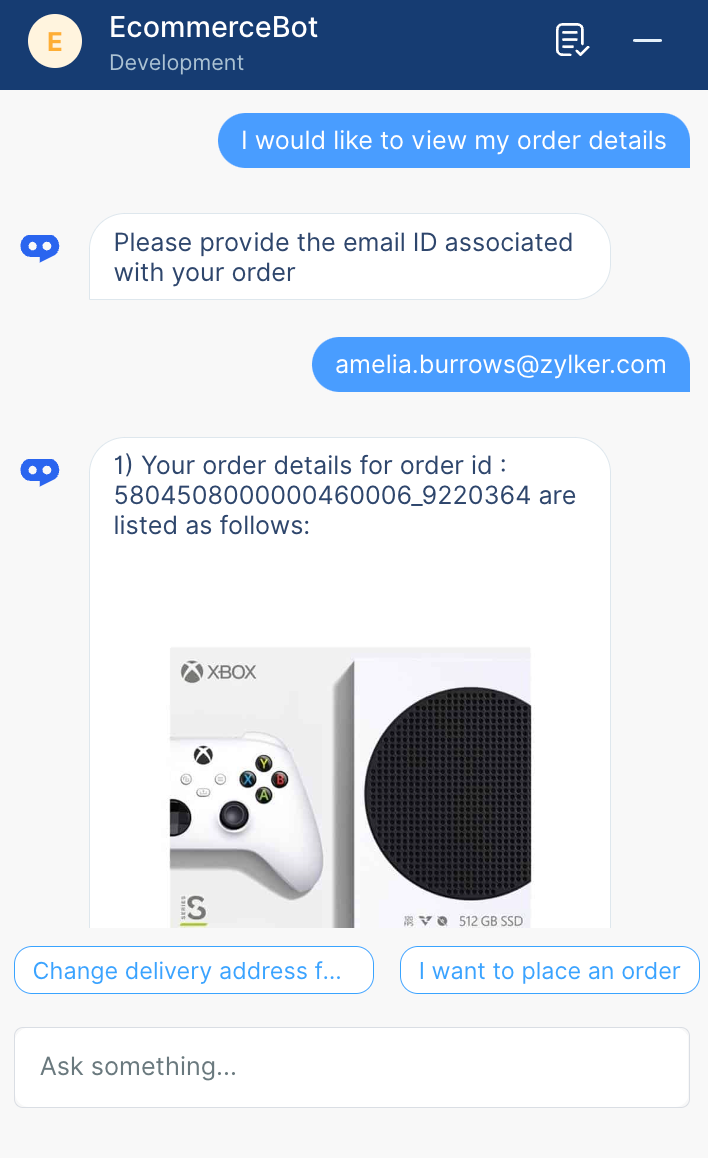This is a screenshot of a chat interface featuring an e-commerce chatbot. The user interface is modern and sleek, with a navy blue bar at the top left corner displaying the text "e-commerce bot" beneath a development label. In the top right corner, the interface includes a minimize line, a list icon, and a check mark symbol. 

The chat itself is designed with alternating message colors: the user's messages are in blue, while the chatbot's responses are in white. The conversation starts with the user saying, "I would like to view my order details." The chatbot responds by asking, "Please provide the email ID associated with your order." The user replies, "amelia.burrows@zylker.com," to which the chatbot responds with, "1. Your order details for Order ID [number] are listed as follows." 

The chatbot provides an image of an Xbox box, which indicates it has "512 gigabytes" of storage. Above the chat bar are two functional buttons: "Change Delivery Address" and "I Want to Place an Order." The chat input field at the bottom prompts the user to "Ask something." The overall background of the interface is light gray, and the design is minimalist with a simple, clean font.